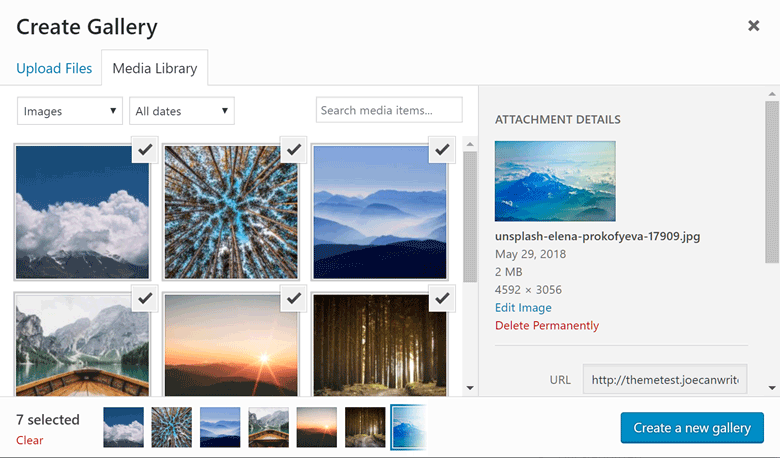A screenshot of a photo gallery creation interface. The background is a clean, white or whitish hue. In the upper left corner, the text "Create Gallery" is prominently displayed in black font. Directly opposite, in the upper right corner, there's a noticeable "X" symbol. Below the top navigation, two clickable tabs are visible: "Upload Files" in blue font and the currently selected "Media Library" in gray font.

Under the "Upload Files" tab, there are two dropdown menus. The menu labeled "Images" is followed by one labeled "All Dates." Between these dropdowns and the main gallery area, a search bar labeled "Search Media Items" is centrally located.

In the main gallery area, six outdoor-themed images are showcased in two rows of three. The images include picturesque shots of clouds, trees, mountains, a sunset, a boat on a mountain lake, and a forest. Each of these six images is selected, indicated by a clear selection overlay.

On the bottom left of the screen, the interface indicates "7 selected," followed by a red "Clear" option. Additionally, thumbnails of the selected images are displayed in a horizontal sequence. On the right-hand side, attachment details for each photo are presented, providing metadata such as date and time taken, pixel dimensions, and options to edit or permanently delete the image.